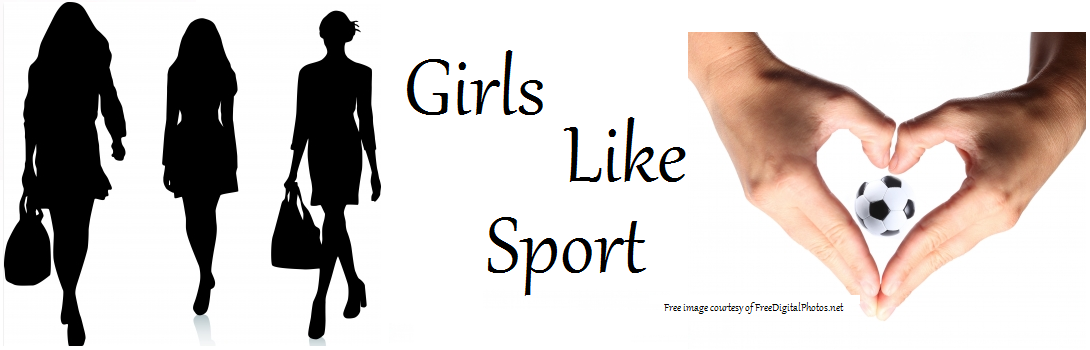This image, in a landscape orientation reminiscent of a banner, features a collection of elements that collectively deliver a message about women and sports. On the left side, there are black silhouettes of three women, all dressed in short skirts or dresses, with two of them – the ones on the outer sides – holding large handbags. These silhouettes depict well-dressed businesswomen, characterized by varying hairstyles: two women with long hair flanking a central figure with short hair. Centrally located text reads, "Girls Like Sport," in bold black on a white background. To the right of the text, two flesh-colored hands form the shape of a heart with their thumbs and forefingers. Inside the heart, there is a black and white soccer ball. Below this image, small text credits the source: “Free Image Courtesy of Freedigitalphotos.net.” This composition suggests a social media meme aimed at promoting the idea that well-dressed women, who are typically seen in professional or casual settings, also enjoy sports. The color scheme is dominated by black, white, and tan, offering a sharp contrast that highlights each element in the image.